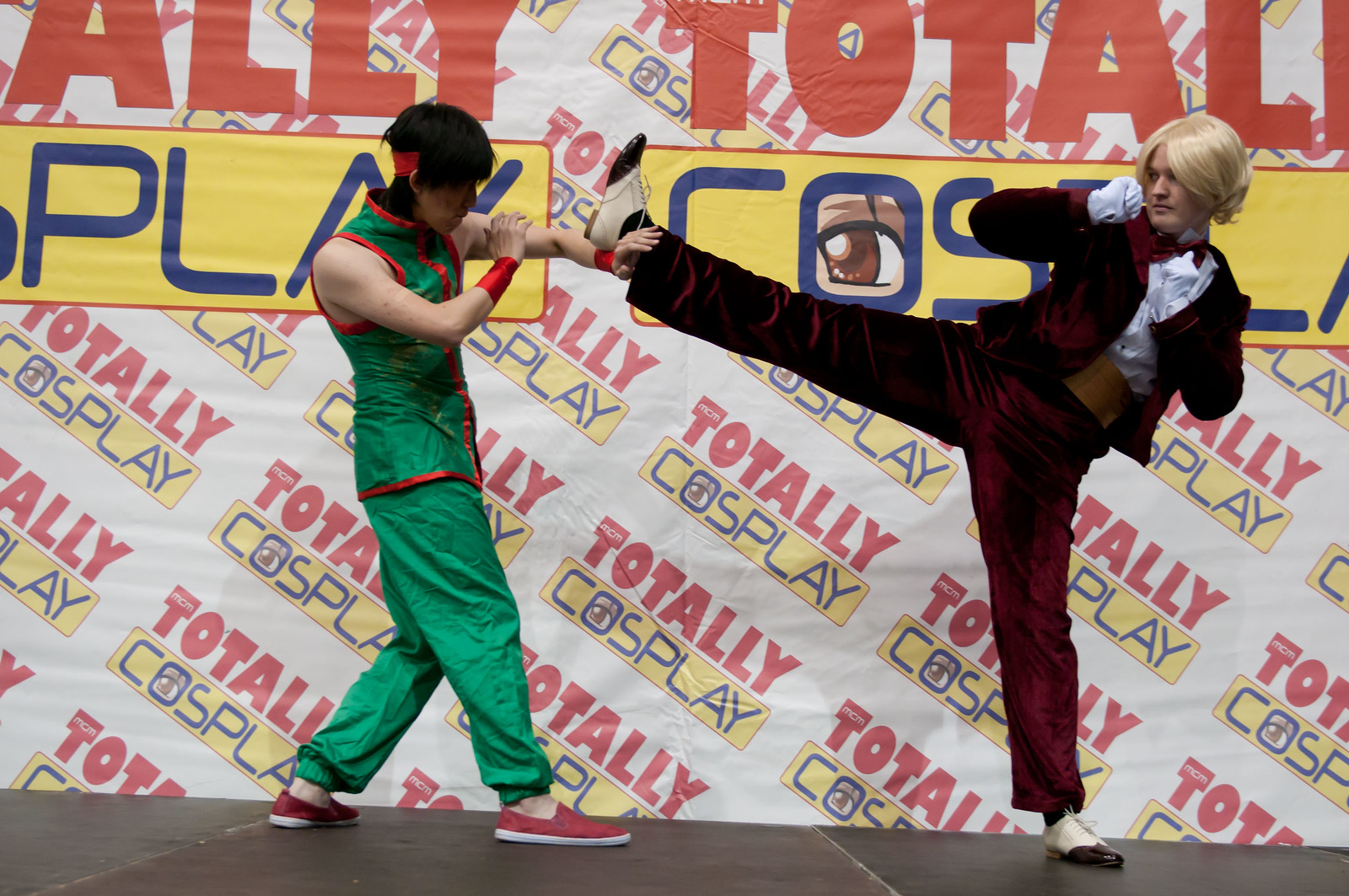The image captures two individuals demonstrating martial arts, possibly karate or a similar self-defense form, on a dark-colored stage at an indoor convention, likely a cosplay event. Both are dressed in elaborate costumes that hint at an Asian martial arts theme. The man on the left, with dark hair, dons a green silk outfit trimmed in red, accessorized with matching red shoes, a headband, and wristbands. He has his hand up in a defensive gesture, blocking a kick from his opponent. The other individual, sporting a blonde wig, is outfitted in a burgundy velvet suit with a white button-down shirt, white gloves, and beige dress shoes. He is mid-kick, with his fists raised near his face. Behind them, a banner that reads "Totally Cosplay" in alternating red and blue letters on a yellow background repeatedly spans the top, set against a white backdrop. The vivid colors of white, red, yellow, and green dominate the scene.